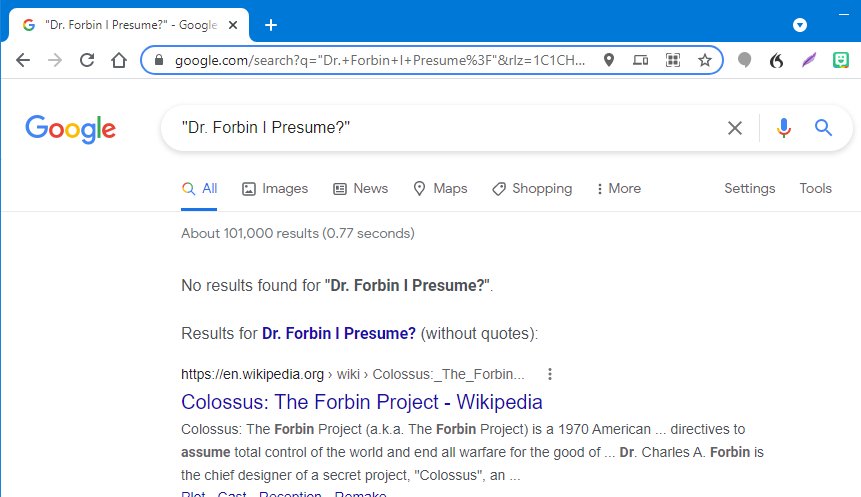The image displays a Google search results page. At the top of the page is a blue bar partially hidden behind the tabs. Below the bar, the well-known Google logo is visible. The search query entered is "Dr. Forbin, I presume," with the entire phrase enclosed in quotation marks. The "All" tab is selected, indicating that all types of search results are being displayed. There are approximately 101,000 results for this query, generated in 0.77 seconds. Despite the number of results, no exact matches for "Dr. Forbin, I presume" were found. Instead, Google has provided results for the phrase without quotes.

The first search result is from Wikipedia and pertains to "Colossus: The Forbin Project," also known simply as "The Forbin Project." This 1970 American film involves directives aimed at assuming total control of the world to end all warfare. The highlighted text mentions Dr. Charles A. Forbin, who is the chief designer of the secret project named "Colossus." The detailed view of the search results is truncated, but it appears to detail the plot of the film. It remains unclear whether the exact phrase "Dr. Forbin, I presume" is used in the movie. However, the search results strongly suggest a connection to this film.